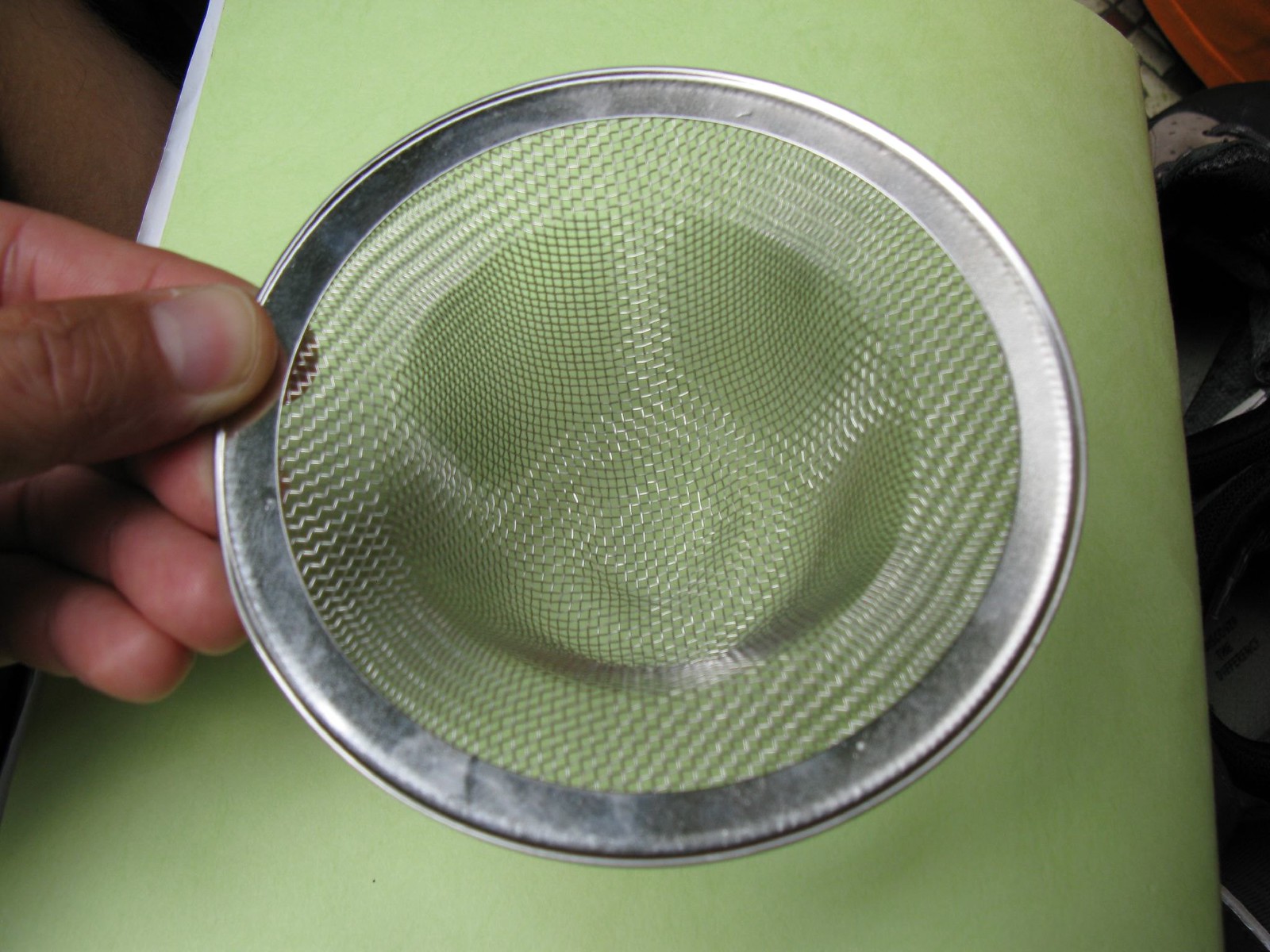The image features a close-up of a hand, with darker colored skin, holding a metal strainer against a pale, seafoam green background. The strainer, which appears to be an aluminum sink strainer, has a thick silver band encircling a mesh wire basket. The strainer is being held in the middle, and its mesh structure appears to be significant in relation to the size of the photo. In the top right corner of the image, there is a brown object, possibly part of a table or plate. Adjacent to this brown object is a shiny black item, which might be an olive or another round object. The green background, possibly a binder or board, adds contrast to the metal strainer and the hand holding it.